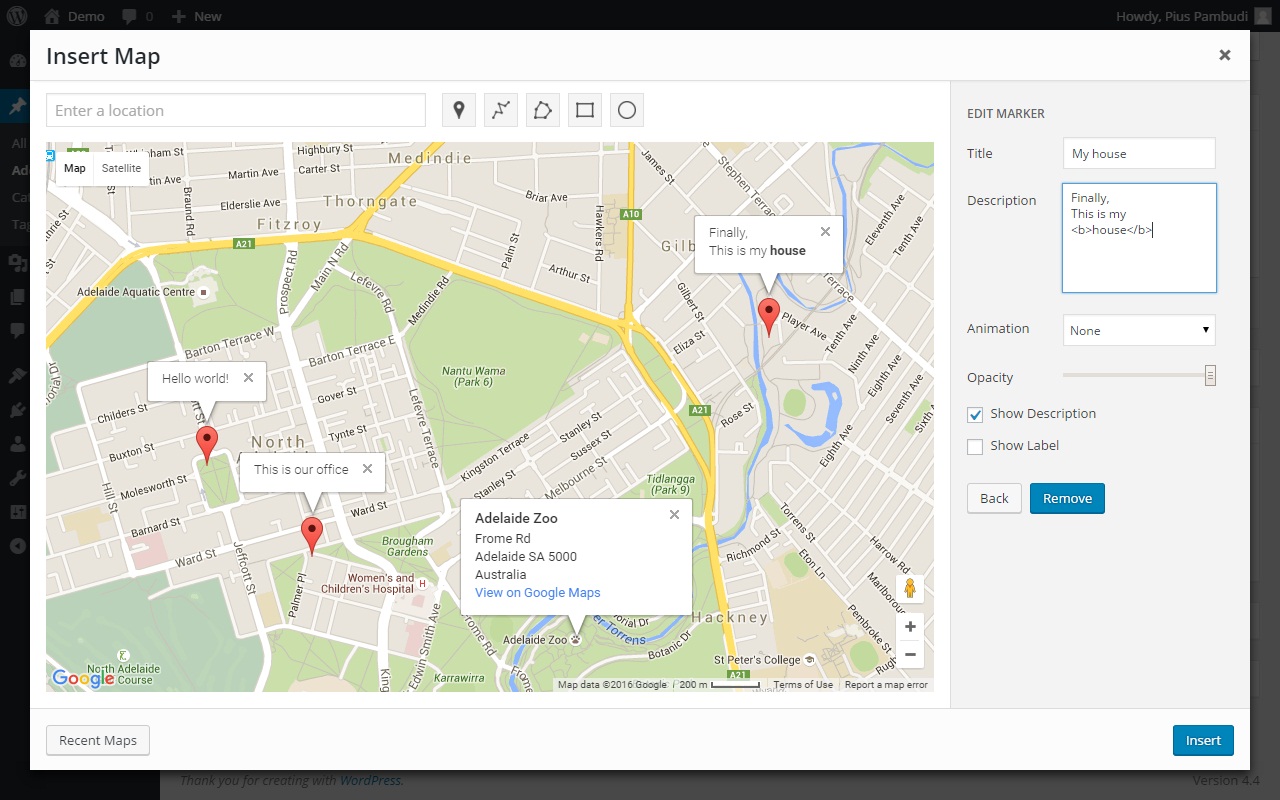The image is a screenshot of Google Maps with a distinctive black border encompassing all four edges. The inner background is light gray, providing a muted contrast. At the top of the screenshot, there's a header that reads "Insert Map," flanked on the right by an 'X' icon for closing the application. Directly beneath this header is a horizontal light gray line that spans the entire width of the image.

Below this line is a prominent text box labeled "Enter a Location," situated on the left. Adjacent to this box on the right is a location pin icon housed within a light gray square. To the immediate right of this setup are four equally spaced squares, arranged horizontally. The far-right square contains a circle icon, while the square immediately to its left contains a solid square icon.

The lower portion of the screenshot depicts an actual segment of Google Maps displaying a top-down view of an area. On the left side, there is a grassy expanse, which transitions into a neighborhood enclosed by an interstate that loops around it. The map details include three red location pins, each with accompanying text boxes. The text box linked to one pin reads "Hello World," while another states "this is our office."